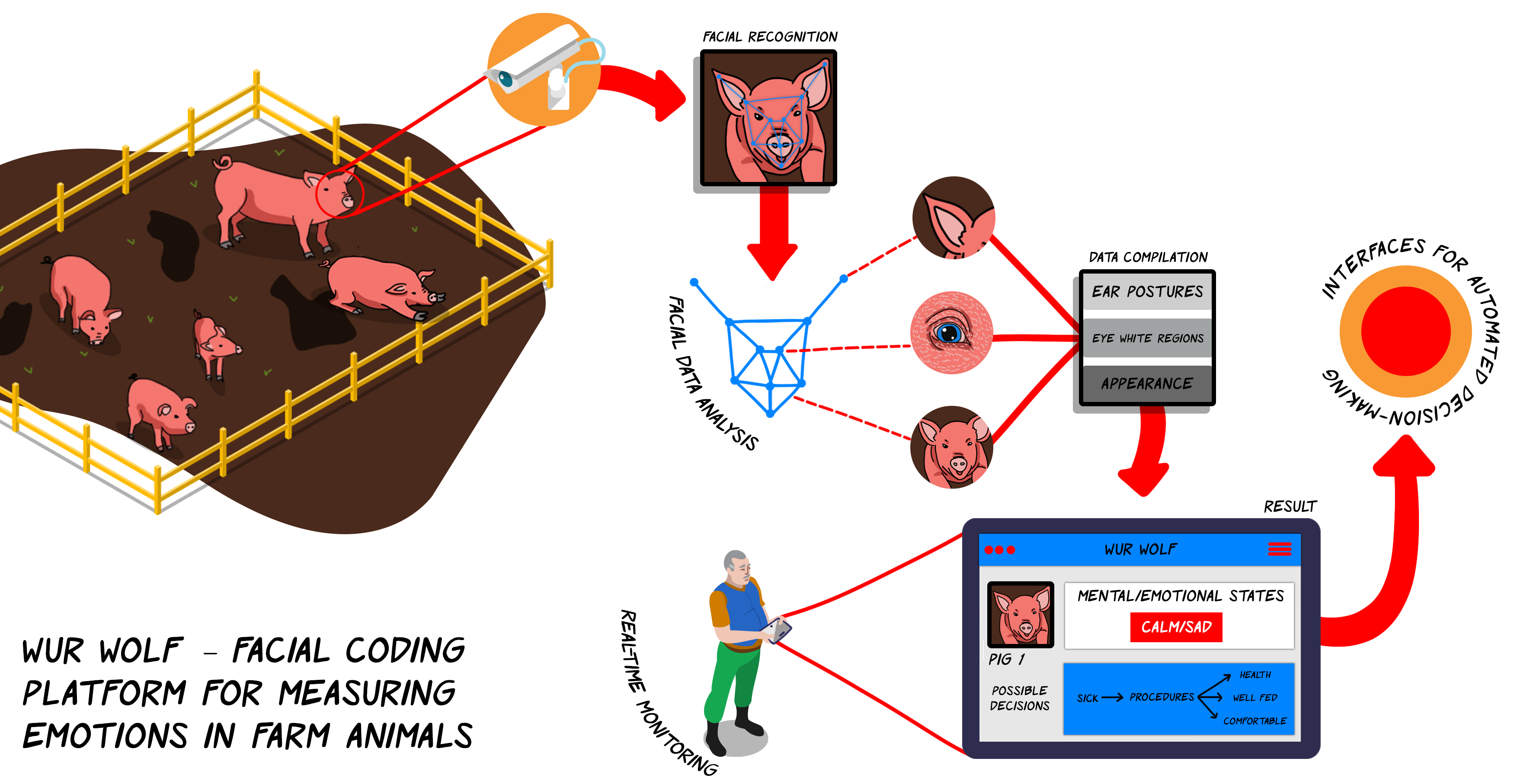This detailed diagram illustrates the Werewolf Facial Coding Platform for Measuring Emotions in Farm Animals. Set against a white background, the main focus is a yellow pen containing five pink pigs of various sizes, standing on a brown, presumably muddy, surface with small green plants. To the left, a camera icon with an orange background is aimed at one pig, highlighted by red lines and a circle around its face. The camera's view leads to an image of the pig's face marked with blue line drawings indicating facial recognition software. Red arrows and lines map out the technology's steps, showing how it analyzes the pig's ears, eyes, and overall facial structure for data compilation. The terms "ear postures," "eye readings," and "appearance" explain the specifics of the software's analysis. All this information is integrated into real-time results, displayed on a tablet held by an older man, demonstrating the platform's capacity for automated decision-making. The bottom left corner of the diagram prominently features the title of the technology: "Werewolf Facial Coding Platform for Measuring Emotions in Farm Animals."